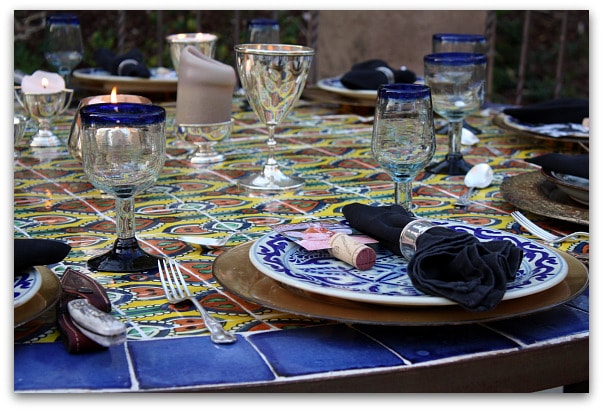This photograph captures a vibrant outdoor dining table adorned with elaborate place settings. The table itself features a stunning design of Italian tiles, with a vivid blue rim and an intricate interior pattern of blue, green, yellow, and a peachy red color in a vague floral motif. Each place setting includes a brown base plate, likely a gold charger, topped with a delicate blue and white intricately designed ceramic plate, possibly transferware china. A blue napkin, secured with a silver napkin ring, is meticulously placed on each setting along with name cards and crackers. To the left of each plate rests a shiny stainless steel fork, accompanied by a partially visible steak knife.

Surrounding the place settings, a variety of clear glasses, possibly water goblets, wine glasses, and chalices, all adorned with blue rims and footings, create a harmonious and sophisticated look. At the center of the table lies a bronze-colored chalice, flanked by a couple of lit candles, casting a warm glow and suggesting a nighttime ambience. The combination of colors, intricate details, and lighting sets a welcoming and festive atmosphere for this dining experience.